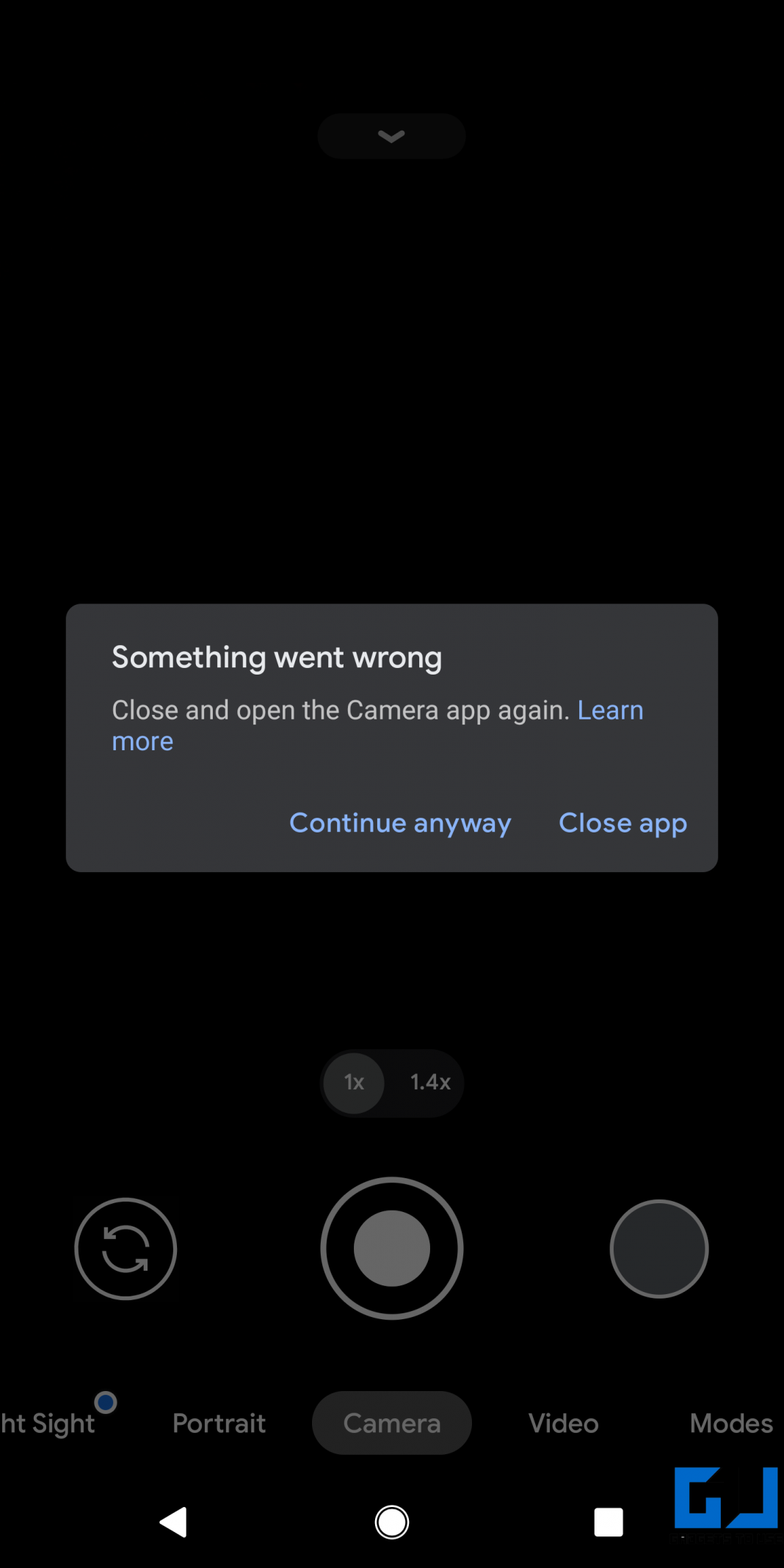The image appears to be a screenshot from a mobile device displaying a malfunctioning camera app interface. The majority of the screen is dominated by a black background, indicating that the camera's live view is inactive. 

At the center of the screen, there's a prominent text bubble that reads, "Something went wrong. Close and open the camera app again." Below this message, there is a hyperlink labeled "Learn more." The user is given two options beneath the hyperlink: "Continue anyway" and "Close app."

Overlaying the camera interface, you can make out familiar icons and buttons. Centered at the very bottom of the screen, partly obscured by the text bubble, are the modes of the camera, partially visible as they are cut off: "Site," "Portrait," "Camera," "Video," and "Modes." Just above these options, the screen shows zoom levels with labels "1x" and "1.4x."

On the left side of the screen, there is a refresh icon, typically used to reset or restart the camera view. The take picture button is prominently located in the bottom center, with a gallery button on the right side for viewing already-captured images.

In the bottom right-hand corner of the screenshot, the letters "GJ" are visible, possibly serving as a watermark or an indicator of the app or device manufacturer.

This detailed screenshot captures the moment when the camera app has encountered an error, demanding user intervention to either rectify the problem or exit the app.